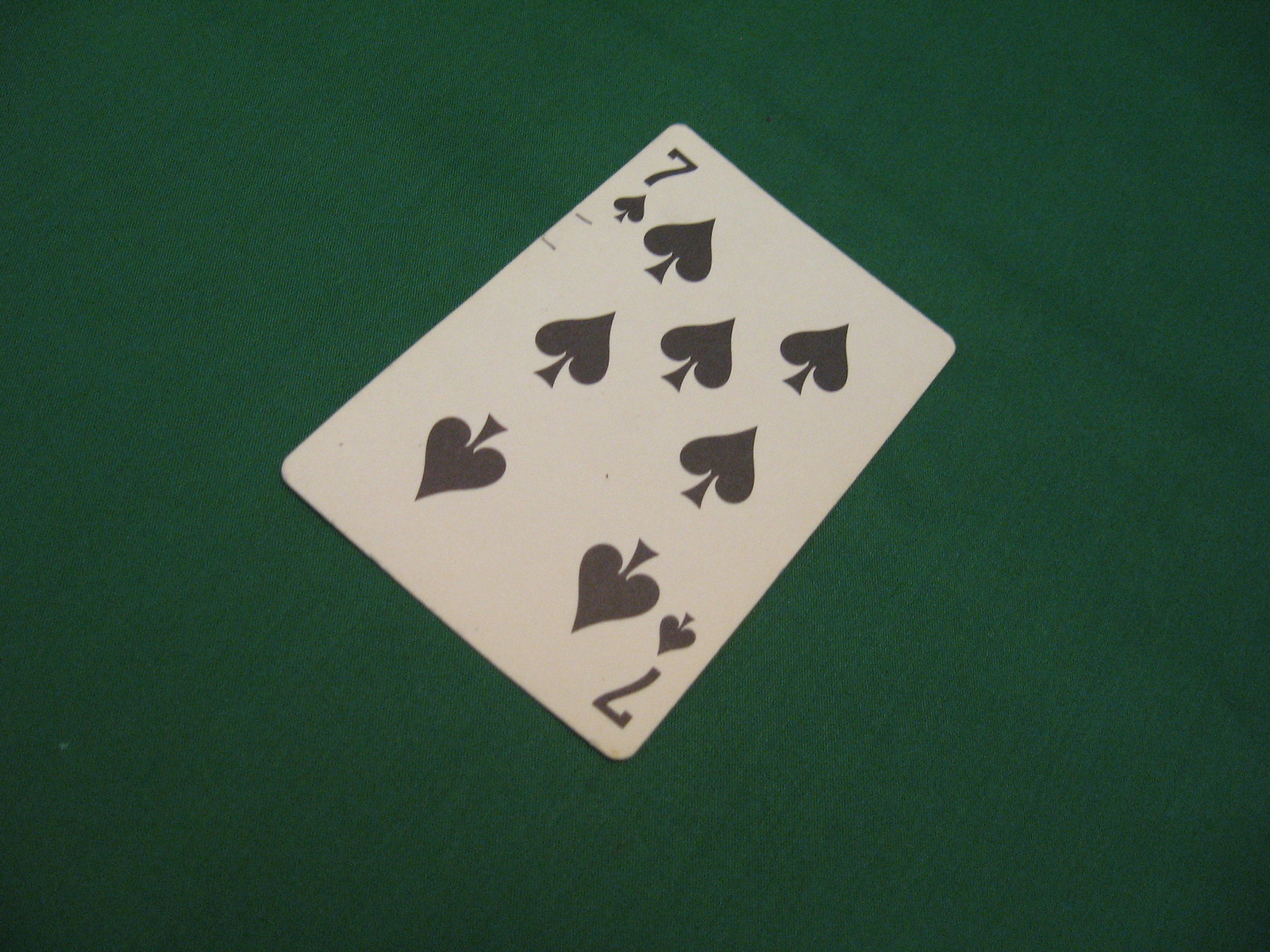The photograph showcases a seven of clubs playing card placed diagonally on a dark emerald green surface. The green fabric background features slight color variations and visible creases, especially towards the bottom two edges, where the shading gives it a darker appearance in the corners. The seven of clubs card, displaying a white backdrop with seven black club symbols, is oriented with its top pointing towards the top right corner of the image. Notably, there are two small scratches or pen marks just beneath the number seven in the top left corner of the card. Despite these minor imperfections and a hint of fading suggesting frequent use, the card remains in relatively good condition.